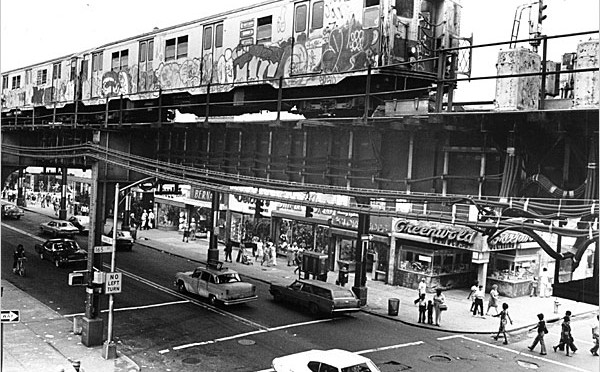This vintage black and white photograph captures a bustling urban street scene, likely from the 1970s or 1980s. Prominently featured above the city street is an old-fashioned, blocky subway train with two cars, completely covered in graffiti, running from left to right on an elevated railroad track. Below, the street teems with activity: numerous cars, reminiscent of mid-to-late 20th-century vehicles, fill both lanes of traffic going in opposite directions. Pedestrians crowd the sidewalks, with many walking across the street, adding to the bustling atmosphere. On the left side of the image, a cyclist navigates down the road towards the center. This commercial area is flanked by several storefronts, and a green-walled store marks the corner. This industrial setting, laden with signs of urban life, encapsulates a vivid snapshot of city dynamism and architectural design from a bygone era.